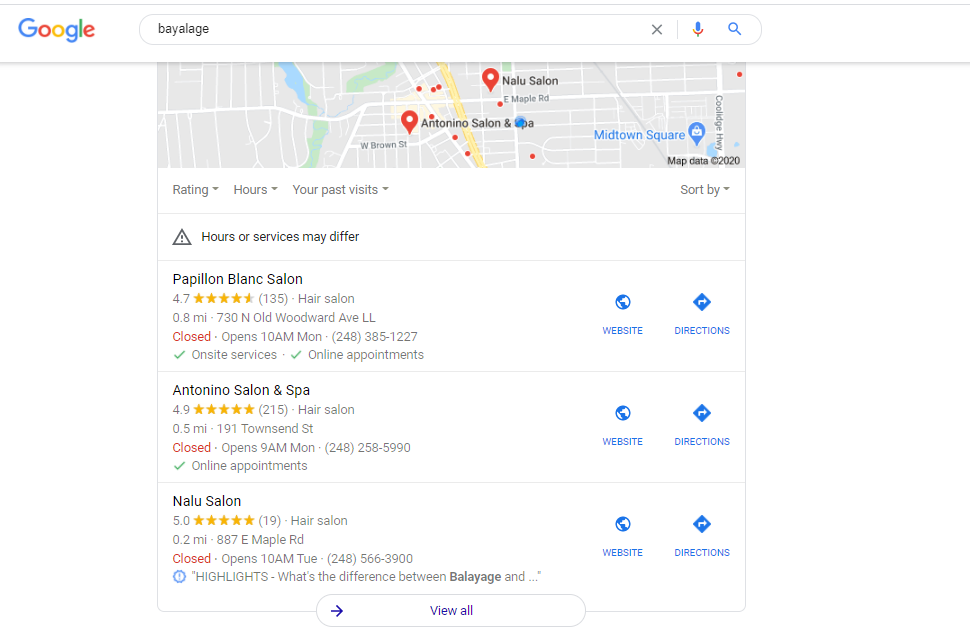The image is a screen capture of a Google search results page for "Balayage." At the top, the classic Google logo appears with its combination of blue, red, yellow, and green letters. Below the logo, there is a white search box containing the term "Balayage" with a gray 'X' for clearing the text, and to the right, a blue and red microphone icon for voice search, as well as a blue magnifying glass icon for initiating the search.

The screen shows a partial map from Google Maps, displaying two red location pins indicating Nalu Salon and Antonio Salon and Spa. A blue dot marks the user's location near Antonio Salon and Spa, with the area labeled as Midtown Square. The map also includes the note "map data © 2020."

Below the map, there are various filtering options in gray text: "Ratings," "Hours," and "Your past visits," all accompanied by pull-down menus. Additionally, there is a triangle icon with an exclamation mark, alerting users that "hours or services may differ."

The first set of business listings features several hair salons, each highlighted with specific information:

1. **Papillon Blanc Salon**
   - Rating: 4.7 stars from 135 reviews
   - Type: Hair Salon
   - Distance: 0.8 miles
   - Address: 730 North Old Woodward Avenue, LL
   - Status: Closed, opens 10 a.m. Monday
   - Phone: 248-385-1227
   - Services: On-site services, online appointments
   - Additional: Links to "Website" and "Directions"

2. **Antonio Salon and Spa**
   - Rating: 4.9 stars from 215 reviews
   - Type: Hair Salon
   - Distance: 0.5 miles
   - Address: 191 Townsend Street
   - Status: Closed, opens 9 a.m.
   - Phone: 248-258-5990
   - Services: Online appointments
   - Additional: Links to "Website" and "Directions"

3. **Nalu Salon**
   - Rating: 5 stars from 19 reviews
   - Type: Hair Salon
   - Distance: 0.2 miles
   - Address: 887 East Maple Road
   - Status: Closed, opens 10 a.m. Tuesday
   - Phone: 248-566-3900
   - Additional: Links to "Website" and "Directions"

Below the listings, the screen partially shows an article titled "What's the difference between balayage and..." with a "View all" link in a white box with a blue arrow.

This detailed breakdown provides insights into nearby salons offering balayage services, complete with their ratings, distances, addresses, hours of operation, and contact information.